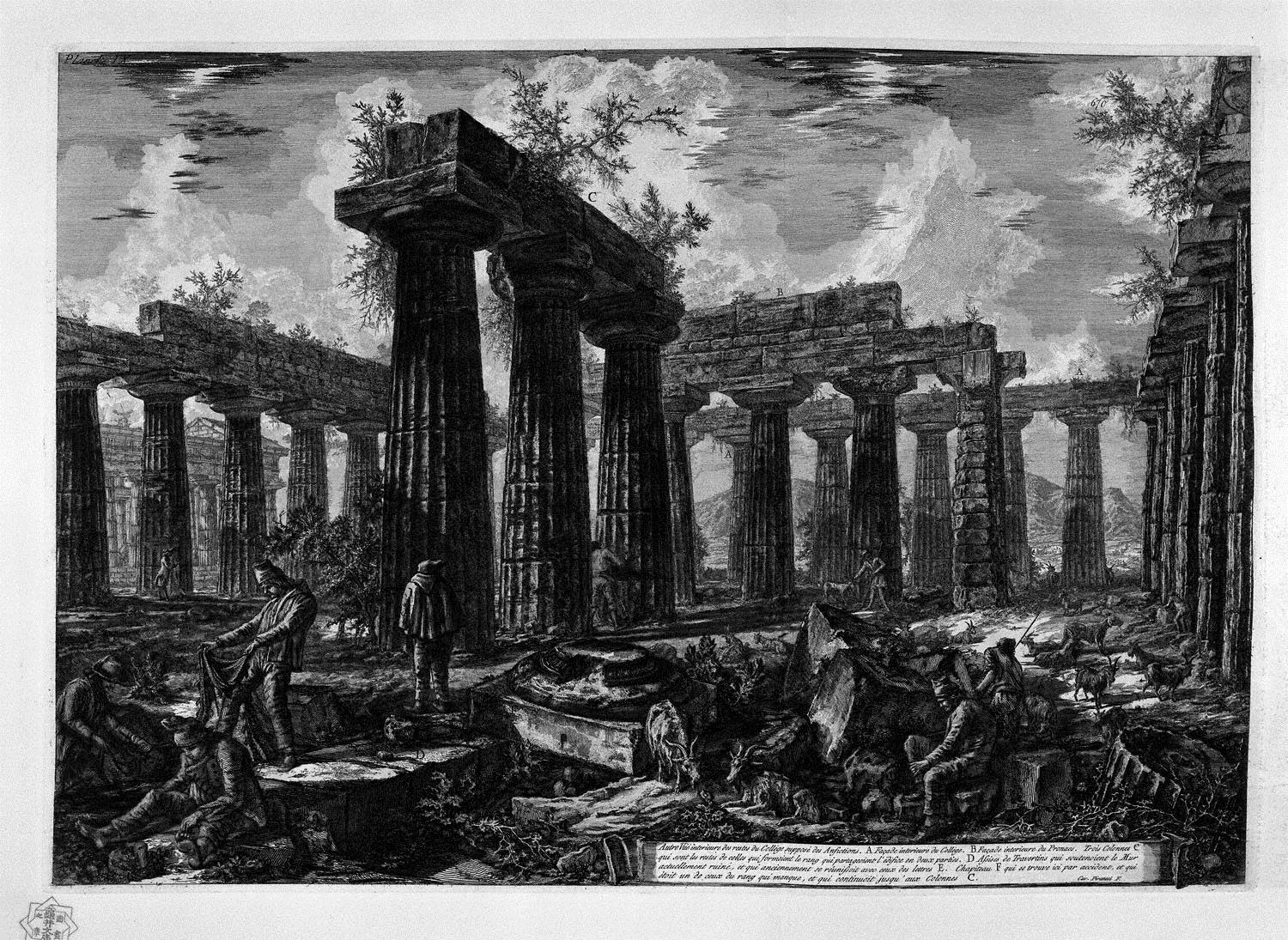This is a highly detailed black and white painting, possibly a computer-generated sketch, depicting the ruins of an ancient structure surrounded by towering Roman columns. The once grand building is now mostly collapsed, leaving only a few pillars that dominate both the right, left, and central parts of the image. At the top of these ruinous columns, plants have begun to take root, adding to the sense of abandonment and decay. The sky above is an ominous, active expanse, filled with large, dark clouds indicative of a stormy or overcast day. 

In the foreground, there are several people, who appear engaged in various activities, possibly working or cleaning around the ruins. Some of these figures are standing, while others are sitting, creating a scene bustling with subdued human activity. Scattered among the people are a few goats, which look malnourished, adding a stark note of hardship to the image. 

The painting features a detailed, light grey border that frames the entire scene. In the bottom right corner of the painting, there is a text box filled with small, cursive script, although the exact wording is indiscernible due to its size. The combination of element details, shading, and the use of black and white gives the overall scene a somber and historic feel.